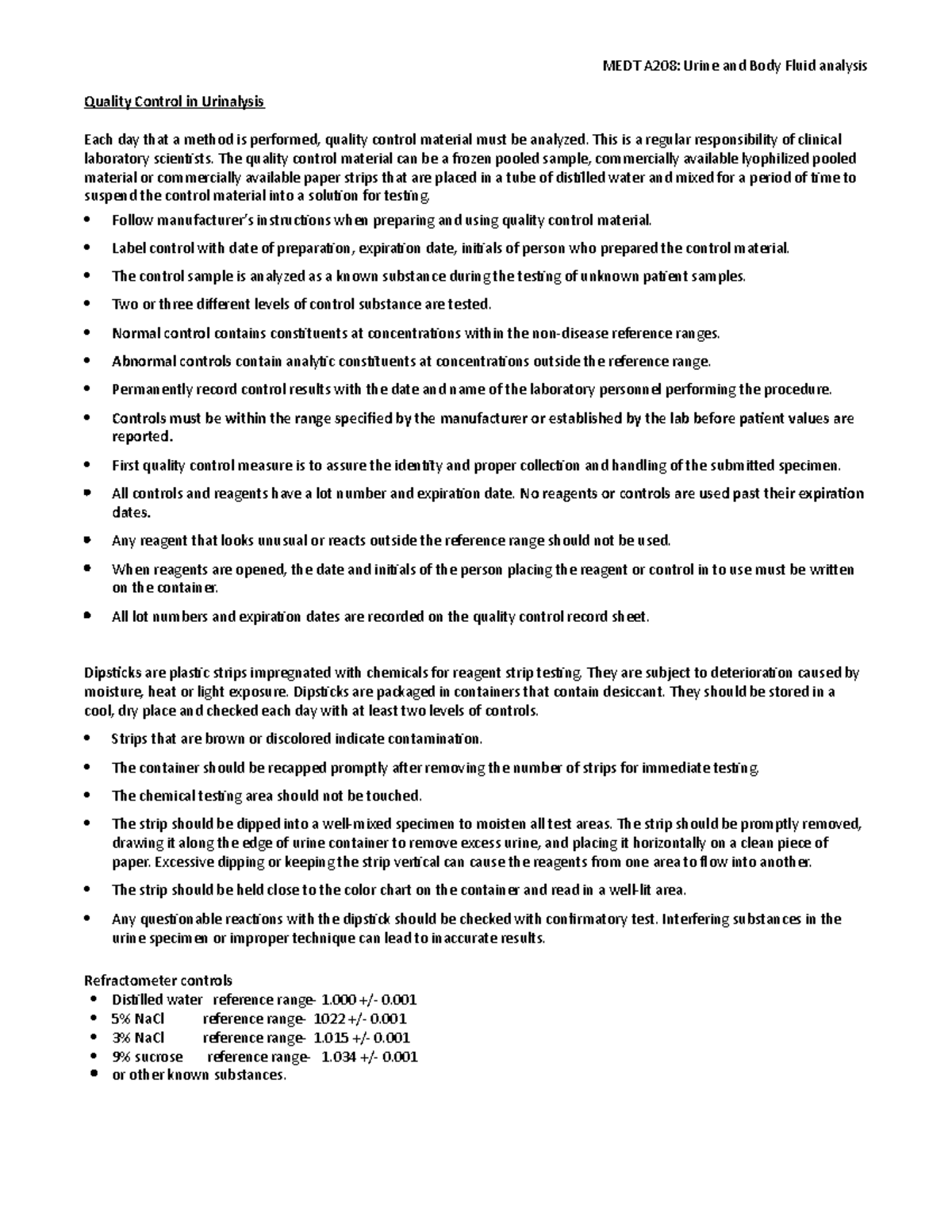This is a detailed screenshot primarily consisting of black text on a white background. The text includes varying levels of boldness and displays information related to "Quality Control Urinalysis." It outlines that each day a specific method is performed, it is mandatory to conduct a quality control analysis. This is a standard responsibility for clinical laboratory scientists. 

The text details 12 protocols for analyzing dipsticks, which are plastic strips embedded with chemicals used for reactant strip testing. There are also 8 protocols specified for refractor controls, including the use of distilled water, 5% and 3% nitric acid, and sucrose. Additional text refers to "Med AE, 20A, Urine and Body Fluid Analysis."

The structured presentation and varying boldness indicate that this text likely serves as a procedural or instructional guideline for laboratory personnel.